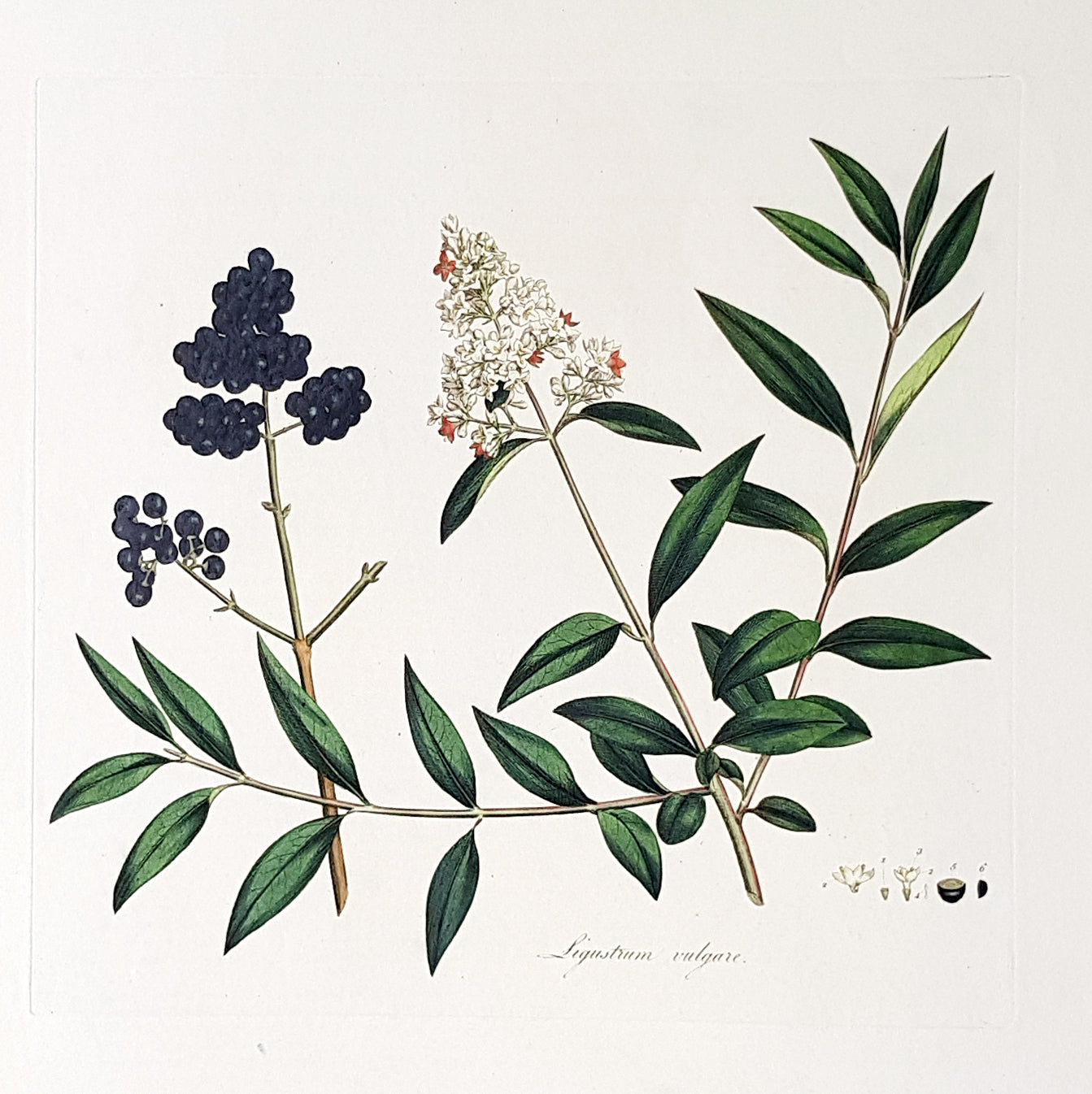In this illustration, twigs and stems extend from the bottom to the top of the image, set against a light blue background. On the left side, a branch prominently features blueberries at its top. On the right, a branch splits into multiple smaller branches with lush green leaves, some extending across the bottom left, while another shoots upward to the upper right. The main stem veers towards the upper left, ending in clusters of small white flowers arranged in a triangular shape. In the central part of the image, there's a distinct white flower surrounded by different colors, including black, dark blue, green, white, off-white, and touches of coral, with coral-colored buds on it. At the bottom, two words are inscribed in black script, though they are difficult to decipher. The style of the illustration hints at it being either a hand-drawn piece or a meticulously created digital print, with scientific accuracy suggested by the textual details.